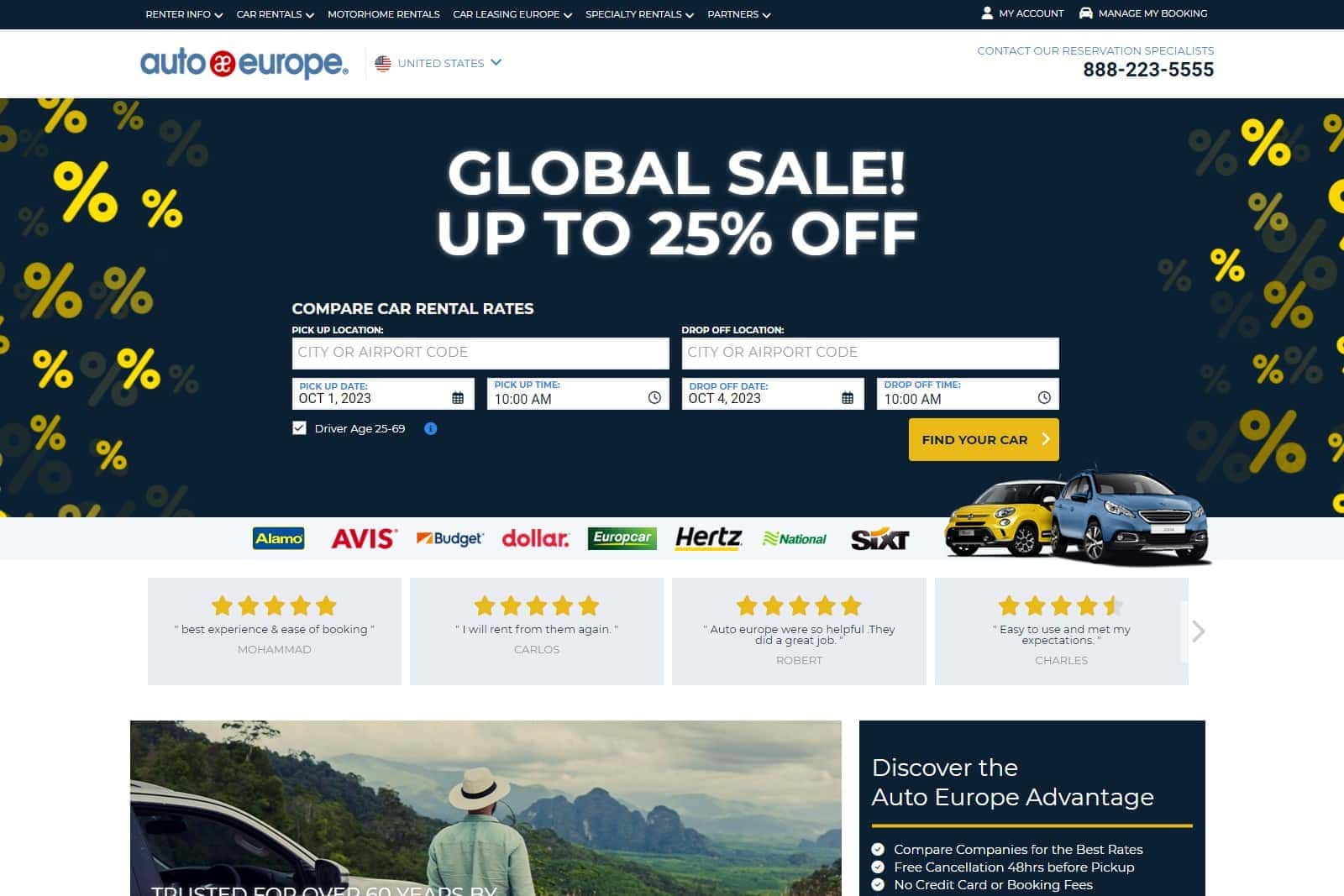In the header of the webpage, starting from the top left, there is a series of drop-down menus labeled: "Rental Info," "Car Rentals," "Multihome Rentals," "Car Lease in Europe," and "Special Rental Partners." On the top right, options for "My Account" and "Manage My Bookings" are available. Below these tabs, the page is titled "Outer Europe," displayed in blue with an icon featuring a red circle and white "AE" in the center. Opposite on the right, the language option "United States" and a contact number for reservation specialists, "888-223-5555," are provided.

The main section showcases a promotional banner stating "Global Sale, up to 25% off" written in white text over a blue background with yellow percentage signs. The search interface prompts users to "Compare Car Rental Rates" with fields for "Pickup Location," "Drop-Off Location," "Pickup Date," "Pickup Time," "Drop-Off Date," and "Drop-Off Time." The driver's age range of "25-69" is pre-checked, and a yellow "Find Your Car" button is situated at the bottom right of the search fields.

Below the search section, two cars, one yellow and one blue, are displayed. To the left, various car rental companies including Alamo, Avis, Budget, Dollar, Eurocar, Europcar, Hertz, National, and Sixt are listed along with their ratings. Three of these companies boast five-star ratings, visually represented by yellow stars. User reviews feature prominently: Mohamed praises the "Best Experience and Ease of Booking," Robert appreciates Auto Europe as "so helpful" with a "great job," and Charles rates it 4.5 stars, stating it is "easy to use and meets my expectations."

At the bottom, an image of a person standing on a mountain is accompanied by text declaring Auto Europe has been "Trusted for over 60 years by." On the right side, the benefits of choosing Auto Europe are highlighted under "Discover the Auto Europe Advantage," with key points including "Compare companies for the best rate," "Free cancellation for hours before pickup," and "No credit card or booking fees," all written in white text against a blue background.